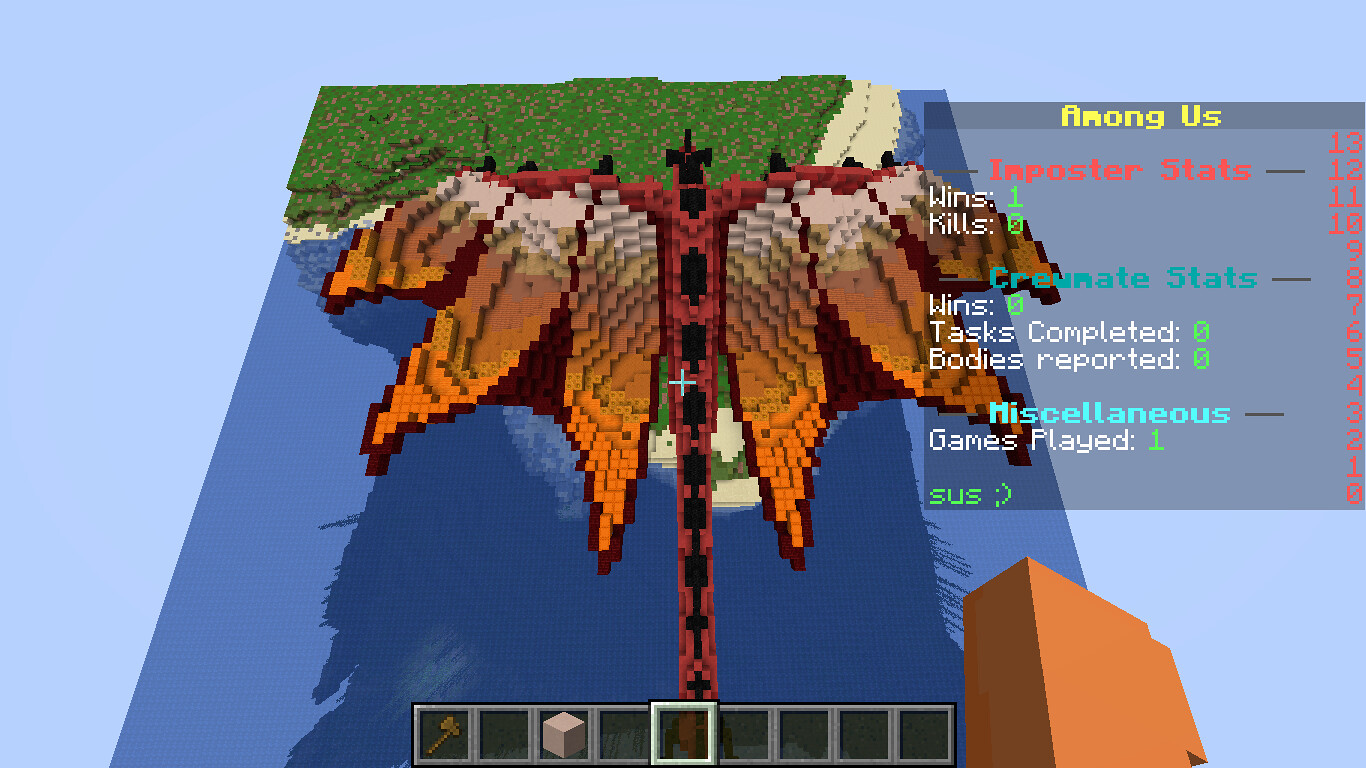This screenshot from a retro-styled video game features a pixelated display reminiscent of 1980s or early 1990s graphics. The main background is light blue. In the upper right corner, there is a slightly darker blue transparent square containing game statistics. At the top, "Among Us" is written in yellow, and below it, "Imposter Stats" is displayed in red. The stats include various numbers ranging from 13 down to 0, detailing wins and kills labeled in white, with "1" for wins and "0" for kills. Additional stats such as "crewmate stats" indicating wins, tasks completed, and bodies reported, all marked as zero, are also present alongside miscellaneous details showing games played and a playful "sus" with a winky face in green at the bottom.

Dominating the center of the image is a pixelated creature that could be described as either a giant bug or a dragon. It has a brown and black segmented body with light brown or tan wings divided into three sections. This creature appears to be flying over a landscape that includes a sandy beach and green grass or forest, with blue water representing the ocean in the background. On the lower right-hand side, there's a brown building near the shoreline, adding to the scene's detailed setting.